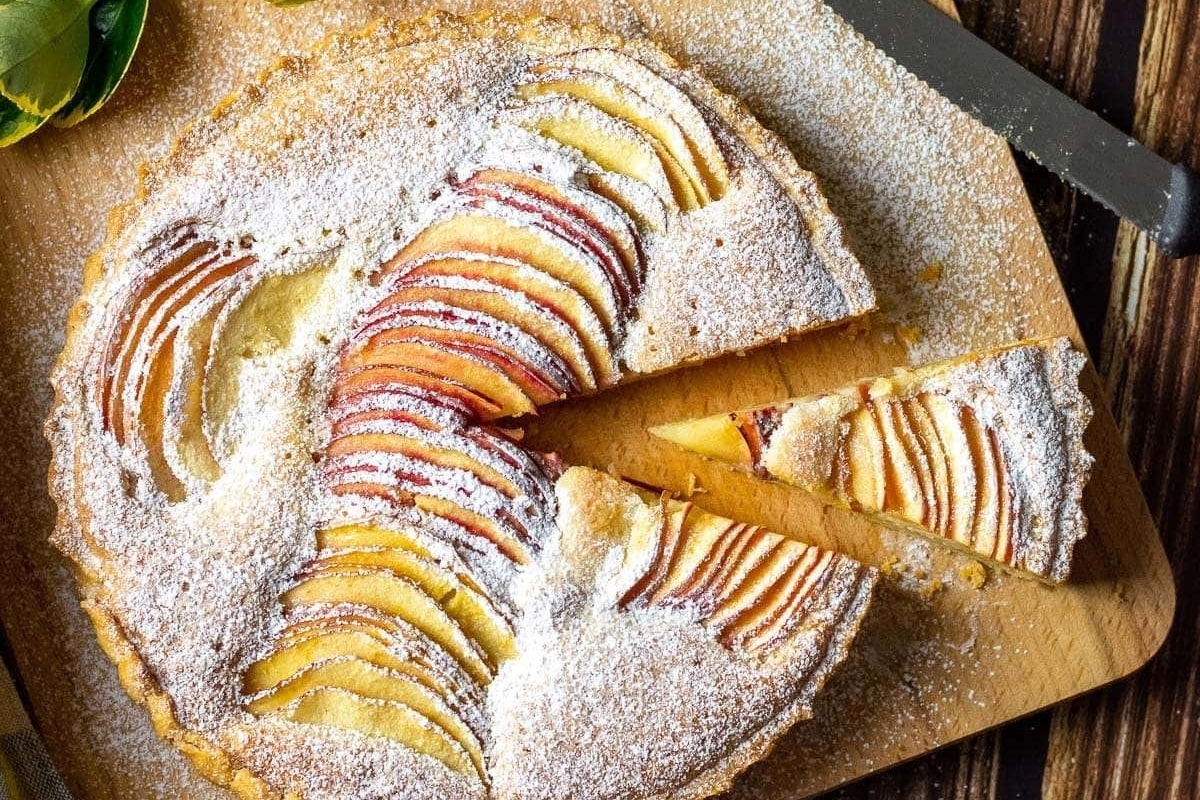The image depicts a freshly baked apple pie with a crusty, perforated texture, resting on a wooden cutting board. The pie is adorned with apple slices arranged to form an X shape on top, each slice generously dusted with powdered sugar. Sprinkles of sugar have also scattered onto the cutting board. A single slice has been cut from the pie and is positioned to the right, next to a knife likely used for the task. The scene is set against a wood grain table, adding rustic charm. In the upper left corner of the image, some leaves tinged with yellow and green can be seen, adding a touch of natural color to the arrangement.